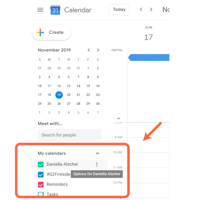The image depicts a serene outdoor scene with a predominantly blue sky. Near the top of the image, there is a small, irregularly-shaped element that captures attention. This small section appears to be a distorted white square, where only two of the corners are sharply defined; one corner seems to fold over like a piece of cloth, and another section appears separated by a dark line. The separated portion creates a visual gap displaying a white space, giving the impression of distance or division. Within the small element, green hues dominate, suggesting vegetation or mountain greenery. This green area stands in contrast with the blue background, which includes a small, white, cloud-like formation, further emphasizing the depiction of an outdoor landscape complete with elements of nature and sky.